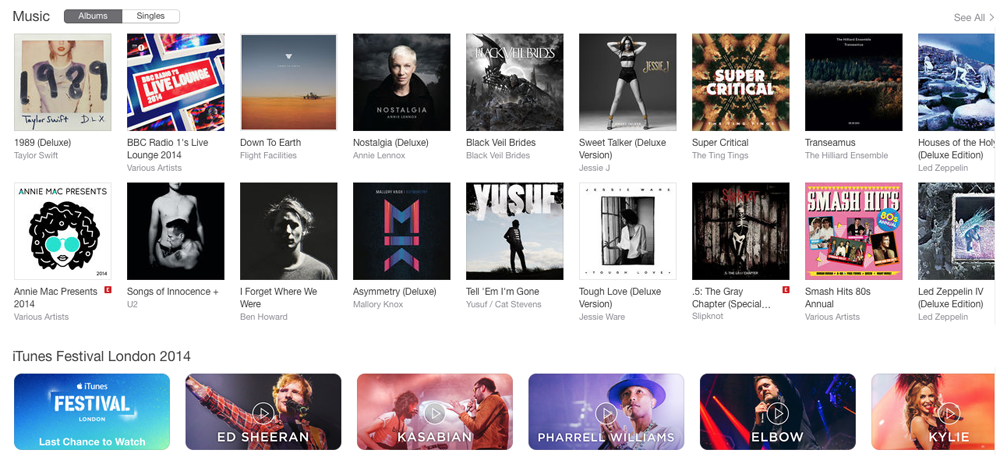Explore the diverse world of music with this eclectic collection of albums and festival performances. Among the highlights is Taylor Swift's "1989 Deluxe" edition, capturing her transition into pop stardom. Tune into the "BBC Radio 1's Live Lounge 2014" for unique live performances. "Down to Earth" by Flight Facilities offers a blend of electronic beats, while Annie Lennox's "Nostalgia Deluxe" brings soulful renditions of classic songs. Rock enthusiasts can enjoy "Black Veil Brides" by Black Veil Brides, and Jessie J's "Sweet Talker Deluxe" delivers powerful pop anthems. The Ting Tings' "Super Critical" injects a dose of indie pop energy, whereas the Hillard Ensemble’s "Trancel Simas" offers a serene classical experience. "Annie Mac Presents 2014" features an array of electronic and dance tunes by various artists.

For rock legends, "Songs of Innocence" by U2 and Ben Howard’s introspective "I Forget Where We Were" are must-listens, alongside Mallory Knox's "Asymmetry Deluxe" for alt-rock vibes. Classic rock aficionados will appreciate the "Led Zeppelin IV Deluxe Edition." Cat Stevens’ "Tell ‘Em I’m Gone" and Jessie Ware’s "Tough Love Deluxe Version" add richness with their distinct styles. Slipknot fans can delve into "The Gray Chapter Special Edition." For an '80s flashback, "Now That’s What I Call Music 80s Annual" offers a nostalgic compilation.

Lastly, the "iTunes Festival London 2014" features unforgettable live performances from artists like Ed Sheeran, Kasabian, Pharrell Williams, Elbow, and Kylie Minogue. This collection spans genres and eras, providing something for every musical taste.